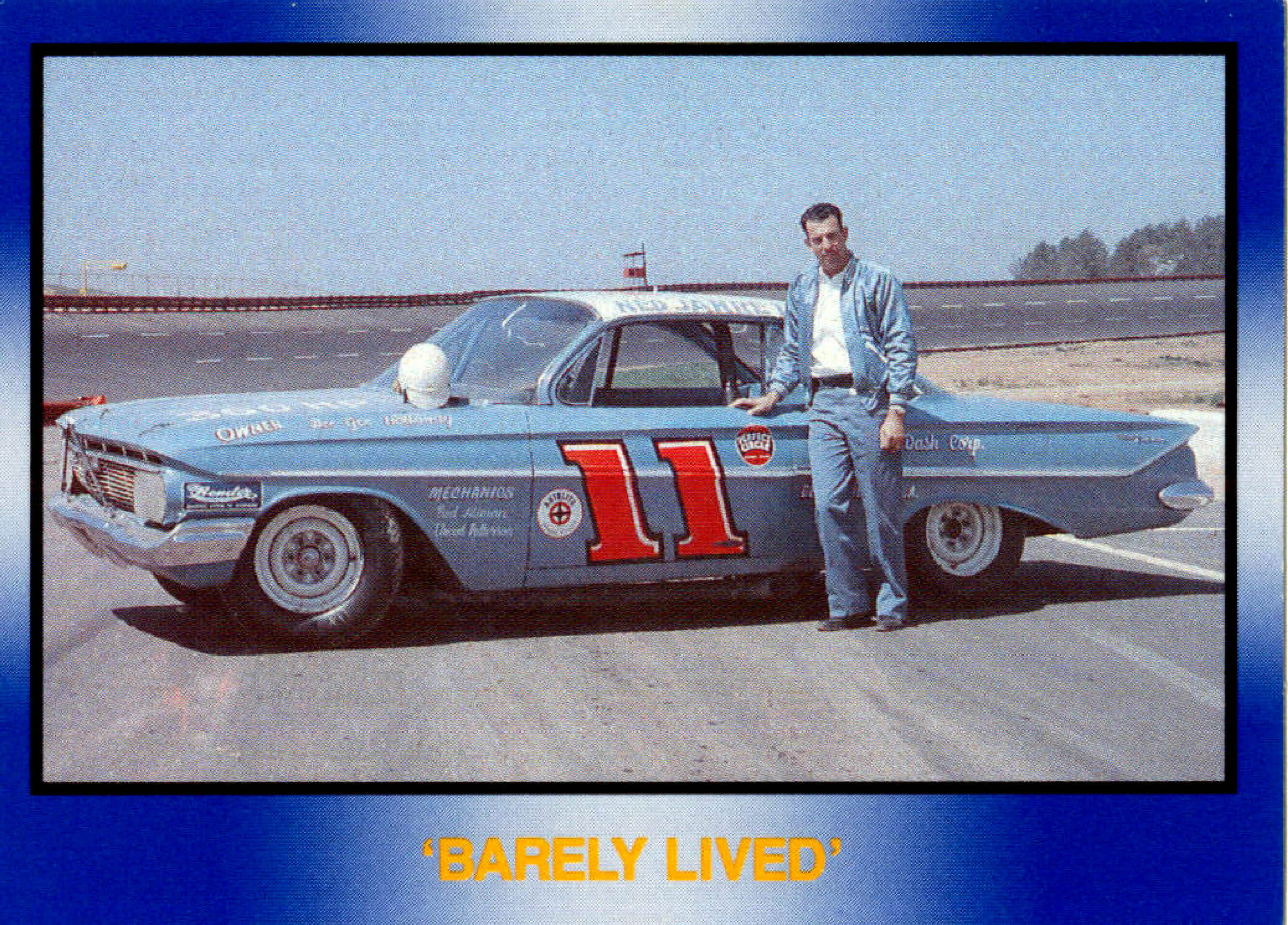This is a wide rectangular photograph encased in a digital frame with a thick dark blue border that fades into a silvery white color on each side. The frame is especially thick at the bottom, where in bold yellow, all-capital letters, it reads "BARELY LIVED." The photograph itself is grainy and has an old-fashioned look. The scene is set next to a gray road in the background, which serves as the horizon line. A brownish red metal barrier is set against a pale blue sky. In the foreground stands a bright baby blue vintage car, adorned with the number 11 in bold red on its front door and various stickers that might represent advertisements or sponsors. Leaning against the car with his right hand placed on it is a man dressed in blue to match the car. He wears a blue jacket, a white shirt underneath, and blue jeans, and has short dark hair. The photograph encapsulates a nostalgic moment, with the man posing confidently before what appears to be a classic race car.